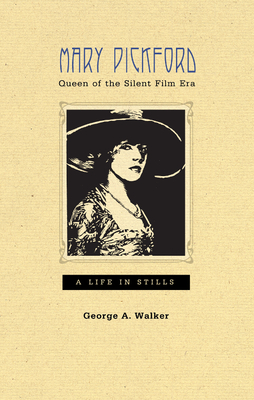This is the cover of a vintage book titled "Mary Pickford, Queen of the Silent Film Era." The background is a tannish or light yellow color. The cover's design features a large, black rectangular frame in the center, containing a black and white illustration of Mary Pickford. She is wearing a low-cut, patterned dress with a floral print, a large necklace, and an oversized hat, which appears to be black. Her pose is turned slightly sideways, facing the camera almost in profile. Above the illustration, the title "Mary Pickford, Queen of the Silent Film Era" is printed in a large font. Below the portrait, in a black banner, it reads "A Life in Stills." At the bottom of the cover, the author's name "George A. Walker" is displayed. The print is in blue and black, and the elements are meticulously stacked on top of one another, complementing the vintage aesthetic of the book cover.